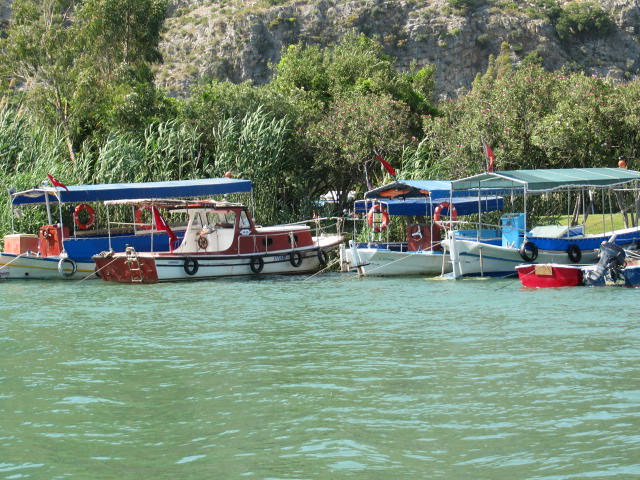A tranquil photograph captures the serene scene of a wide, greenish-blue waterway, with gentle waves covering the entire bottom half of the image. Across the center, from left to right, rests a collection of seven boats near a grassy shore. The boats, which include pontoon types with canvas canopies and simple outboard motorboats, are pulled up towards the shore, not docked. Three of the boats feature distinct canopies: one is green, and two are blue. Several boats display red and white lifesavers on their sides, with some bearing a red flag with white symbols. In the center left, a small houseboat can be observed, adding a quaint touch. In the background, a dense treeline of predominantly green leaves, interspersed with some pink-flowered trees, runs along the shore, gradually giving way to grayish-brown mountains or cliffs with patches of green grass. The scene, bathed in bright daylight suggesting a summer afternoon, underscores a peaceful, picturesque landscape devoid of human activity, as all boats appear stationary and unoccupied.